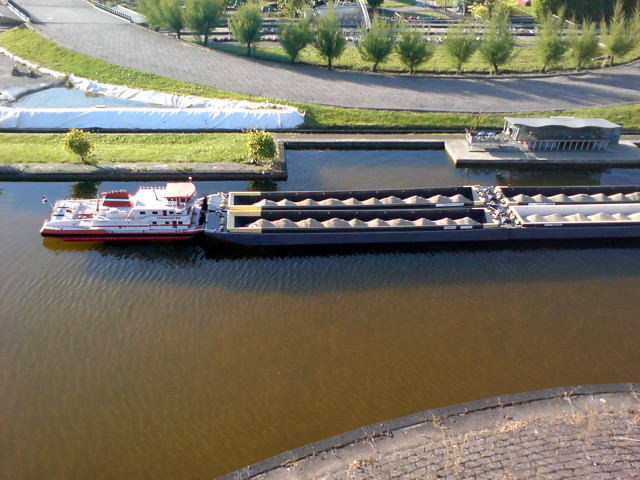In this aerial view, captured from an elevated position possibly from a drone, we see a broad expanse of a brown river that reveals gentle ripples on its surface. Central to the image is a white boat with prominent red and black stripes that is towing a large rectangular barge. The barge is divided into two open sections, each containing pyramid-shaped piles of tan sand, and extends off to the right side of the frame. The boat, positioned to the left, appears to be navigating horizontally across the river.

In the background of the photograph, a gently curving tarmac road arcs through the scene, bordered by lush green grass on both sides. A neat line of dark green trees follows the contour of the road, adding to the picturesque landscape. On the lower right section of the image, a grey cobblestone pavement interspersed with brownish plants is visible. To the extreme left and above the river, there’s a small house with a grey roof and a dock with a black roof alongside a surge wall. The scene is bathed in daylight, showcasing the varying textures and colours from the brown water to the vibrant greenery, making it a vivid and detailed capture of this riverside vista.